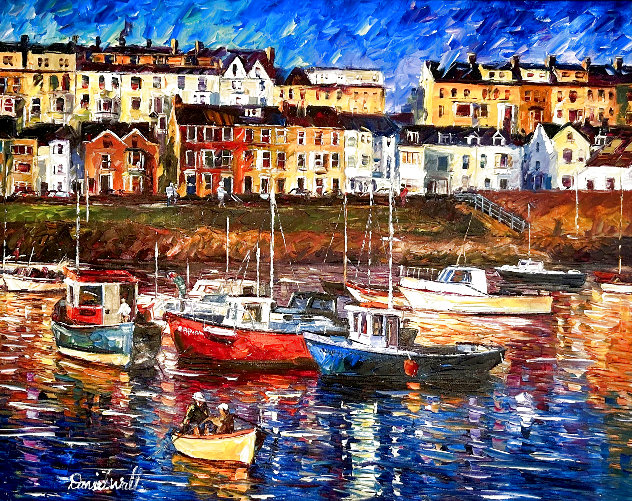The painting "Harbor at Sunset," set in Portugal, captures a serene coastal town scene. In the foreground, a small light brown rowboat with two figures is paddling across calm, reflective waters. Adjacent to this, numerous motorboats in vibrant hues—blue, red, yellow, white, and black—are docked. These vessels, characterized by their sail masts and stocky build, are used by local fishermen. The water, mirroring the sky's vibrant blue tones, enhances the tranquil setting.

In the middle section, a white staircase ascends a green, grassy hill on the right side, leading up to an array of old, multistory European buildings with black roofs. These buildings, painted in shades of white, yellow, red, and tan, form a picturesque backdrop. Smoke rises from some of the chimneys, indicating life within. 

In the distance, factory structures are vaguely discernible, adding a hint of industrial life to the serene town. The brushstrokes are bold and dynamic, capturing the liveliness of the scene while maintaining an overall sense of peace and reflection in the harbor.